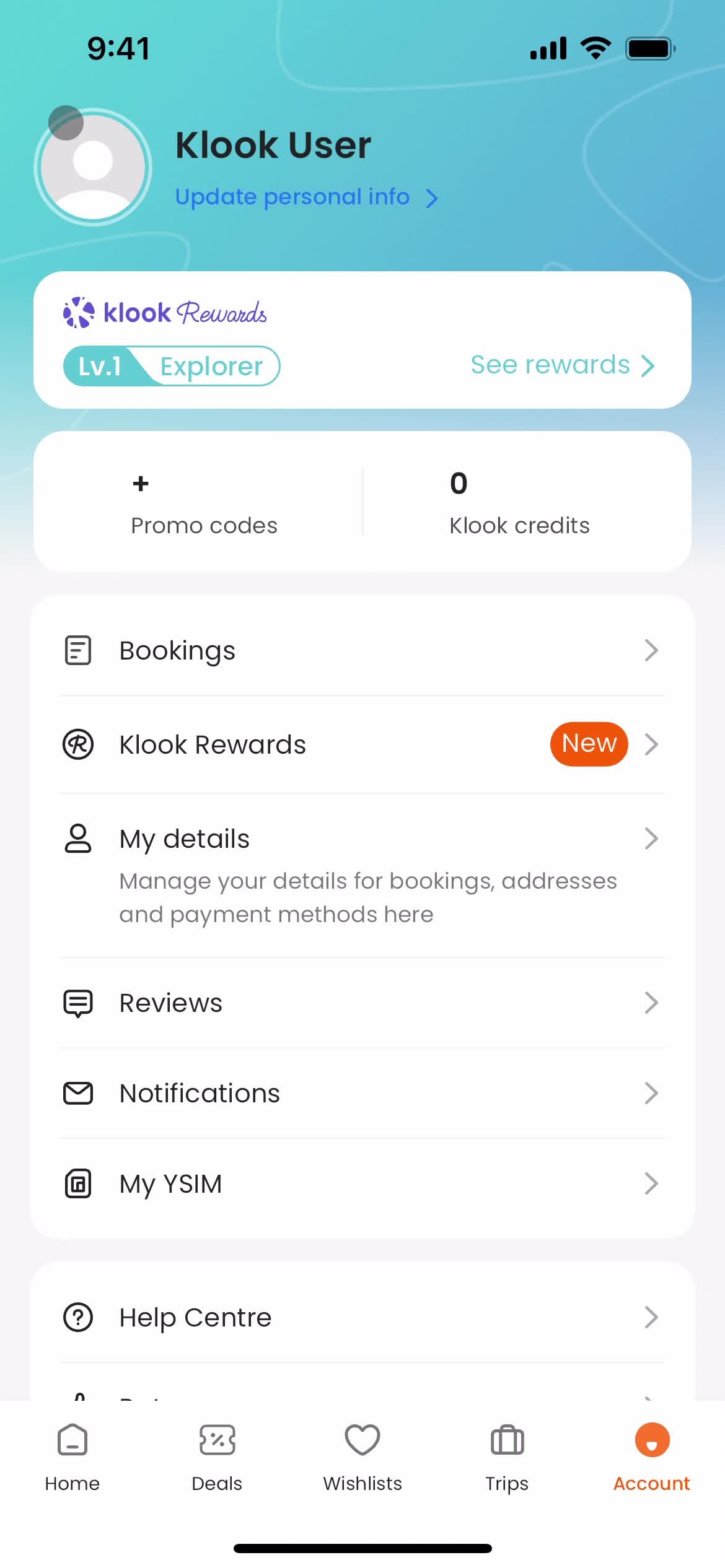This is a detailed picture of a mobile phone screen showing the CLOOK user interface. At the top, against a teal-colored background, the screen displays "CLOOK User" (spelled out as K-L-O-O-K U-S-E-R) along with an option to "Update Personal Info" and a section labeled "CLOOK Rewards." Next to "CLOOK Rewards," there is a clickable teal button that says "See Rewards." Below this, the background transitions to white.

In this white section, there are multiple rows with icons on the left and corresponding text on the right. The first row displays "Bookings." Following that, the "CLOOK Rewards" section appears again, this time with a "New" label in an orange oval. Next is the "My Details" row, which invites users to manage their personal details for bookings, addresses, and payment methods. Below this are sections labeled "Reviews," "Notifications," and "My YSIM." The final row in this section is "Help Center," marked with a question mark icon.

At the bottom of the screen, there is a navigation bar with different icons and labels. From left to right: a house icon beside the label "Home," a coupon icon for "Deals," a heart icon for "Wish List," and a suitcase icon indicating "Trips." The last icon, "Account," is highlighted in orange and features an orange circle above it.